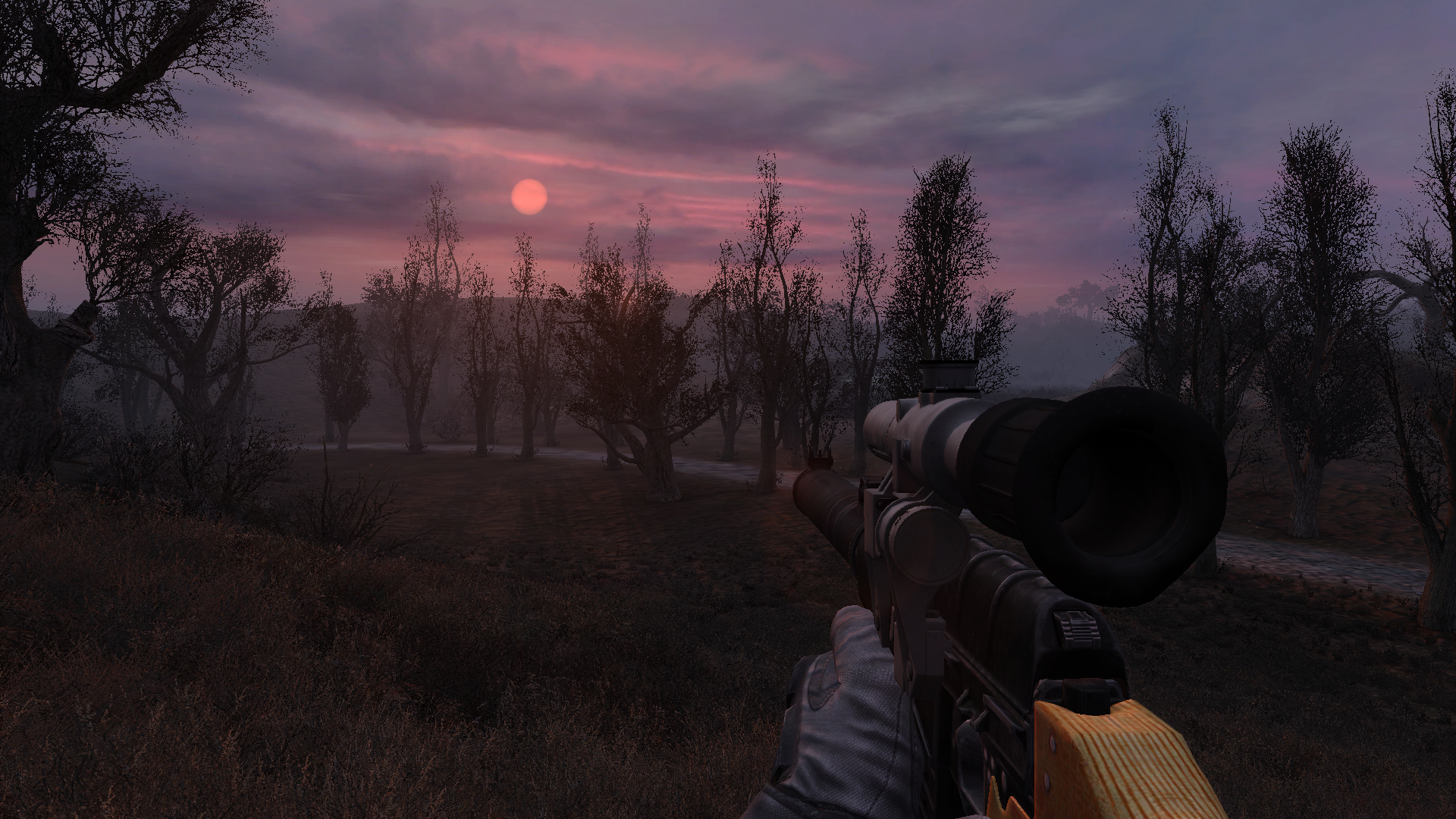In the screenshot from a video game, the player is holding a rifle with a scope, visible in the lower right-hand corner of the view. The player's left hand, wearing a white glove, is grasping the middle section of the rifle, which has a light beige wood handle. The scene captures a dusky, twilight moment, where the faint pink and peach hues of the setting sun cast a subtle glow over the landscape. The sky transitions from a gray-blue to peach near the sun, partially obscured by thin clouds. Silhouetted trees stand on either side of a walking path in the grassy field below, leading to distant, hazy mountains or hills. The overall ambiance is dark and serene, emphasizing the solitary and immersive experience of the player in this virtual environment.